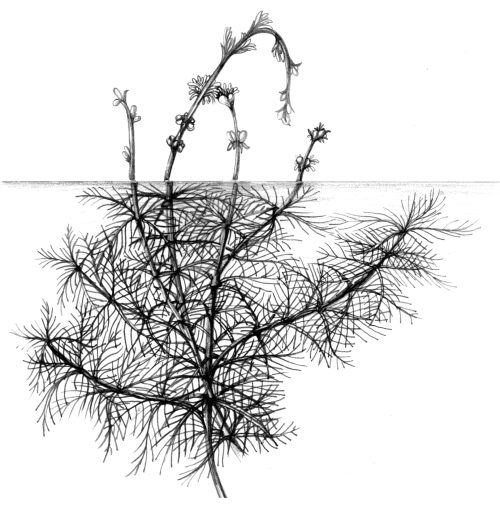The image is a highly detailed black and white drawing of a plant structure. The background is white, highlighting the striking black sketch. A horizontal line slightly above the center divides the drawing into two distinct parts. Below the line, the illustration captures intricate root details, resembling veins or stems intertwined, small and large, akin to fern foliage. Each root extends upward, supporting the main plant structure. Above the line, the plant showcases various flowers and buds. On the left, a three-petaled flower tilts left, accompanied by a two-petaled formation on either side of its lower stem. Adjacent to it, another flower curves like a cane. To the right, additional flowers, some long and tilted, others shorter with multiple petals, complete the elaborate floral display. The entire depiction emphasizes the plant's cellular and vein-like features, portraying its mechanism of water and nutrient transport, entwined with the external beauty of its flowers and buds.